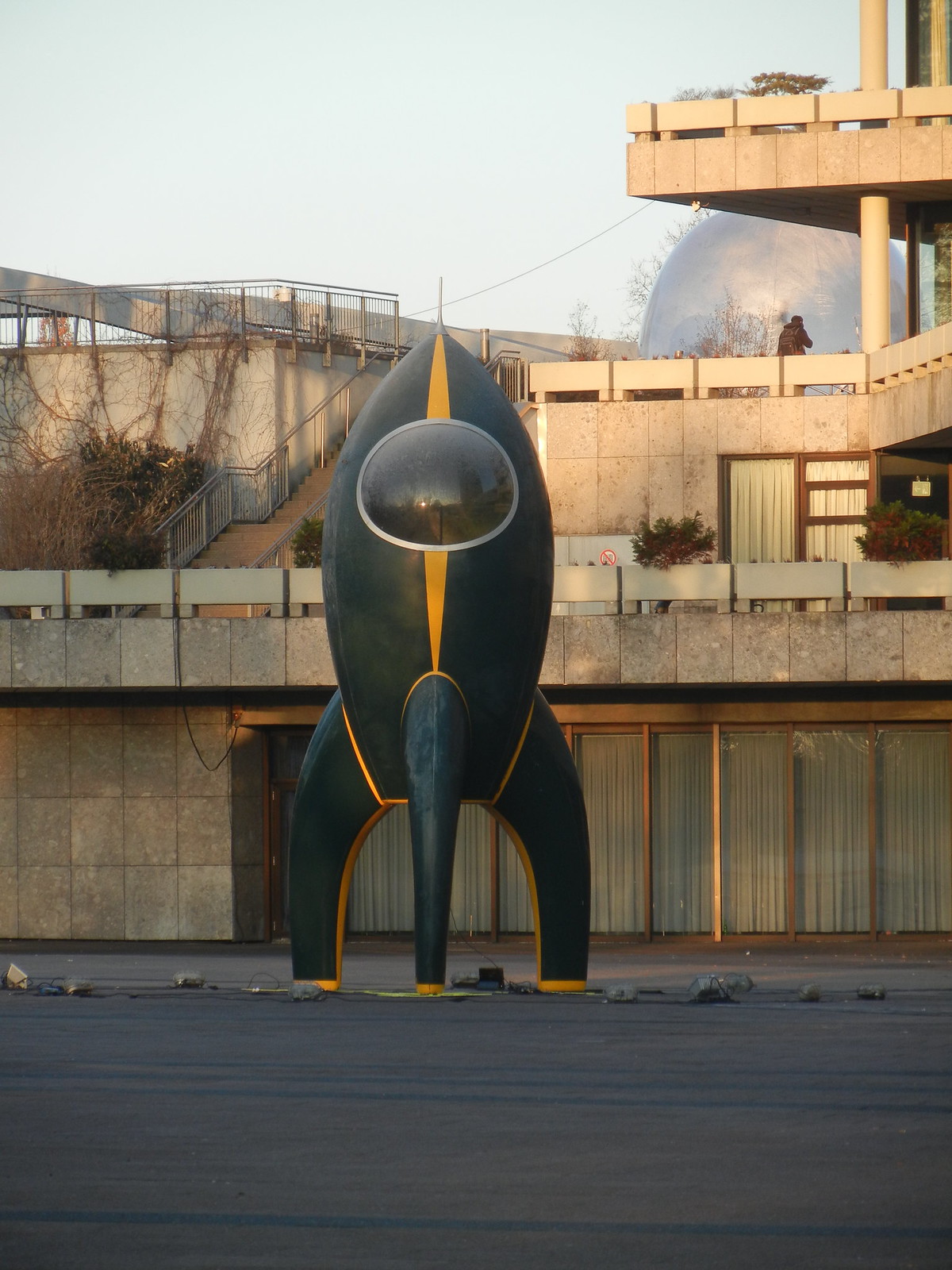The rectangular photograph captures a ground-level view of a scene featuring a meticulously designed modern concrete building in the background. The building showcases a stack of three levels with spacious patio-like balconies, constructed using large, heavy concrete blocks. Each level is lined with floor-to-ceiling windows, framed by stone blocks, and the beige-colored concrete wall builds a sophisticated backdrop. A staircase is visible in the upper left corner, ascending and turning left to connect with another platform extending in a different direction. 

Dominating the foreground is a small, primitively styled rocket ship, painted a dark greenish-black hue with gold and yellow accents. This rocket stands poised on three visible legs, which are black with striking orange borders, giving it a sturdy presence. The rocket’s body is capsule-shaped, tapering to a pointed top. A large, round window reminiscent of a spaceship cockpit is situated in the center of its upper part, suggesting a functional design. The ground beneath the rocket is streaked with dark gray and light blue hues, adding to the space-themed aesthetic. A light blue orb can be seen in the top right of the image, though its purpose remains unclear. The overall impression is that of a display, possibly set up by a space company, as evidenced by the person standing on a balcony and the detailed setting which likely serves as an exhibit for the model rocket.